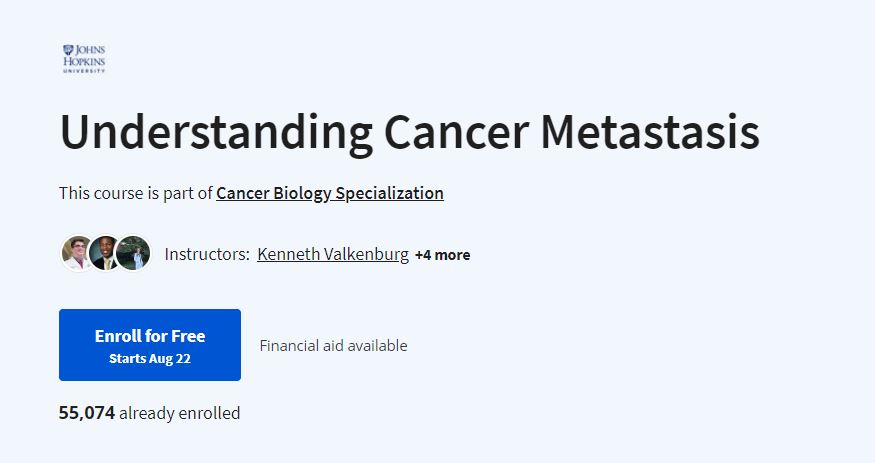This image is a detailed page from Johns Hopkins University, featuring a light blue background with predominantly black text content. In the upper left-hand corner, the name "JOHNS HOPKINS" is displayed in all capital, navy blue letters. Directly beneath it, the word "UNIVERSITY" appears in smaller, navy blue, all-capital letters. Adjacent to the university name is the Johns Hopkins logo or school crest.

The main header of the page reads "Understanding Cancer Metastasis" in large, bold, black text which is also underlined. Below this header, a subheading in smaller, gray letters states: "This course is part of Cancer Biology Specialization."

Beneath the subheading are round profile photos of three individuals, two men and one woman. To the right of these photos, the word "Instructors:" appears in gray text followed by the underlined name "Kenneth Valkenburg." Additionally, the phrase "plus 4 more" is prominently displayed in bold black text.

Below the instructors' section is a bright blue button with bold white text saying "Enroll for Free, Starts August 22nd." To the right of the button, in gray text, it mentions "Financial Aid Available."

Finally, at the bottom of the page, the text "55,074 already enrolled" is displayed, with the number in bold black text and the rest of the text in gray.